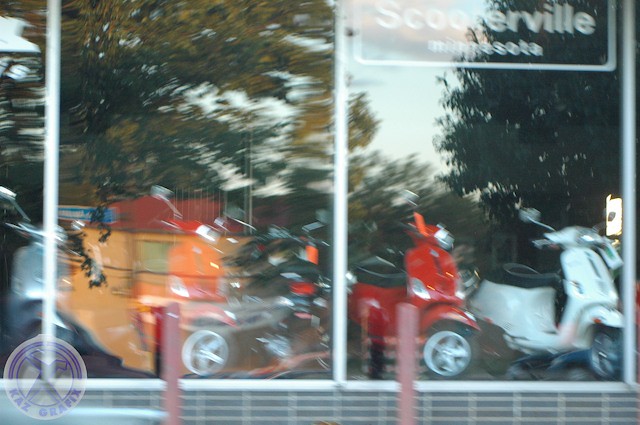This outdoor color photograph, taken from the street, captures a storefront with a clear glass display window that prominently reflects its surroundings. The storefront, identified as Scooterville, features a black sign with white lettering reading "Scooterville" and "Minnesota" below it, positioned in the upper right corner of the window. The window itself is divided into three large panes and rests above a gray block wall. 

Through the slightly blurry glass, a variety of scooters are visible, all aligned and facing to the left. Notably, the scooter farthest to the right is white, followed by a red one, with others partially obscured by reflections. The reflection in the window reveals a yellow building and large, green-leafed trees from across the street. On the right side of the reflection, there's a fluffy tree, and further back, more buildings and trees are discernible. 

Additionally, the image includes scattered elements such as reddish pillars on the street and a logo in the lower left corner with blue lettering reading "CAZ Graphics." The lower right corner showcases a circle with a purple logo, though its text is unreadable. The overall photograph gives a detailed glimpse of both the interior scooters and the external environment through the reflective storefront glass.